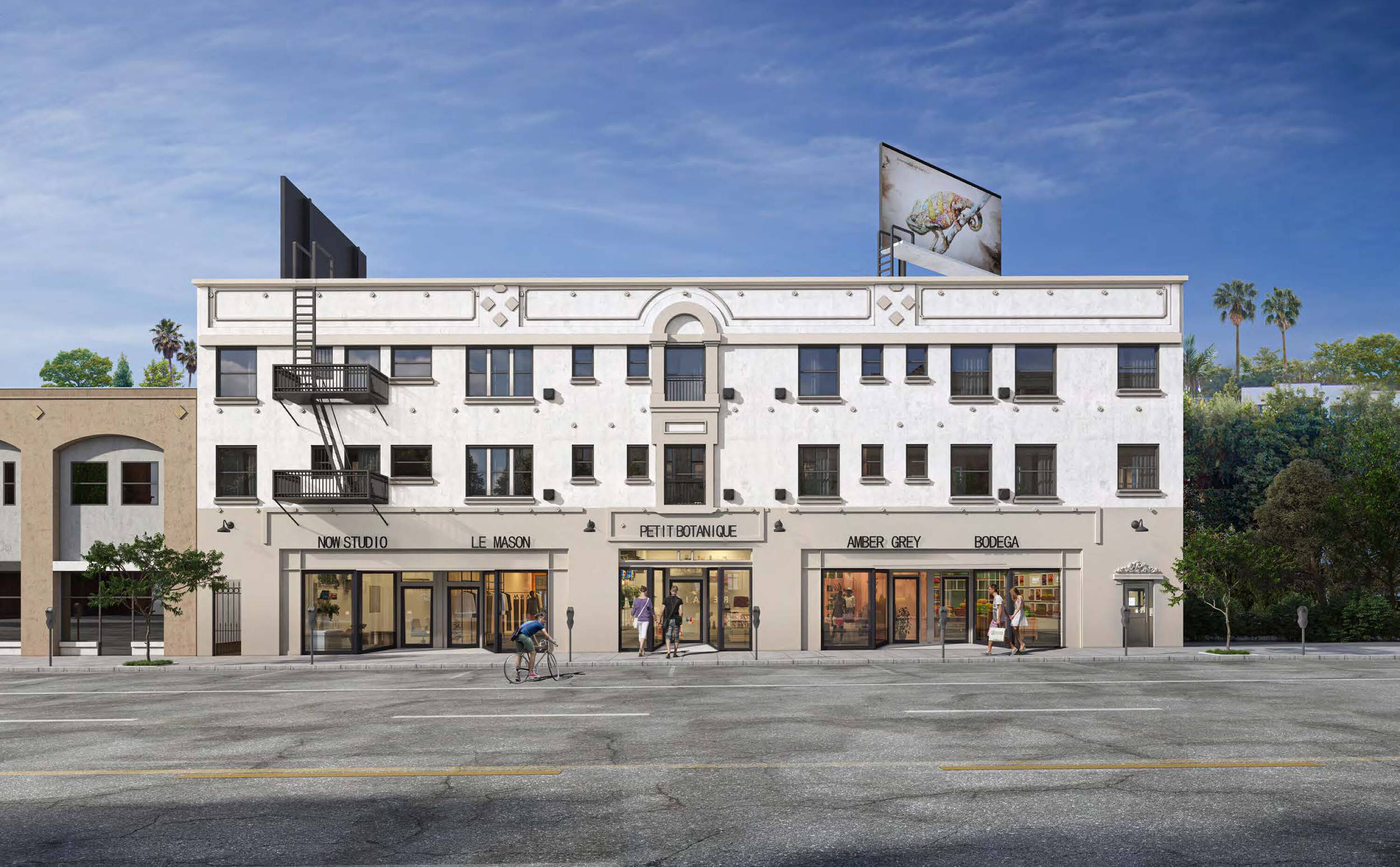This photograph captures a bustling street scene on a sunny day with a light blue sky. Dominating the scene is a white, three-story building with beige accents on the first story, lined with multiple storefronts beneath the two rows of windows. Names in French can be seen atop each storefront, hinting at a shopping area. Adjacent to this building is a two-story brown structure, both framed by small trees and distant tall palm trees, suggesting a Southern California-like environment. A wide four-lane road runs in front, bordered by parking meters and populated with four pedestrians and a bicyclist in a blue shirt. Above the primary building, several billboards rise into the sky, and a sparse scattering of clouds adds depth to the clear day.